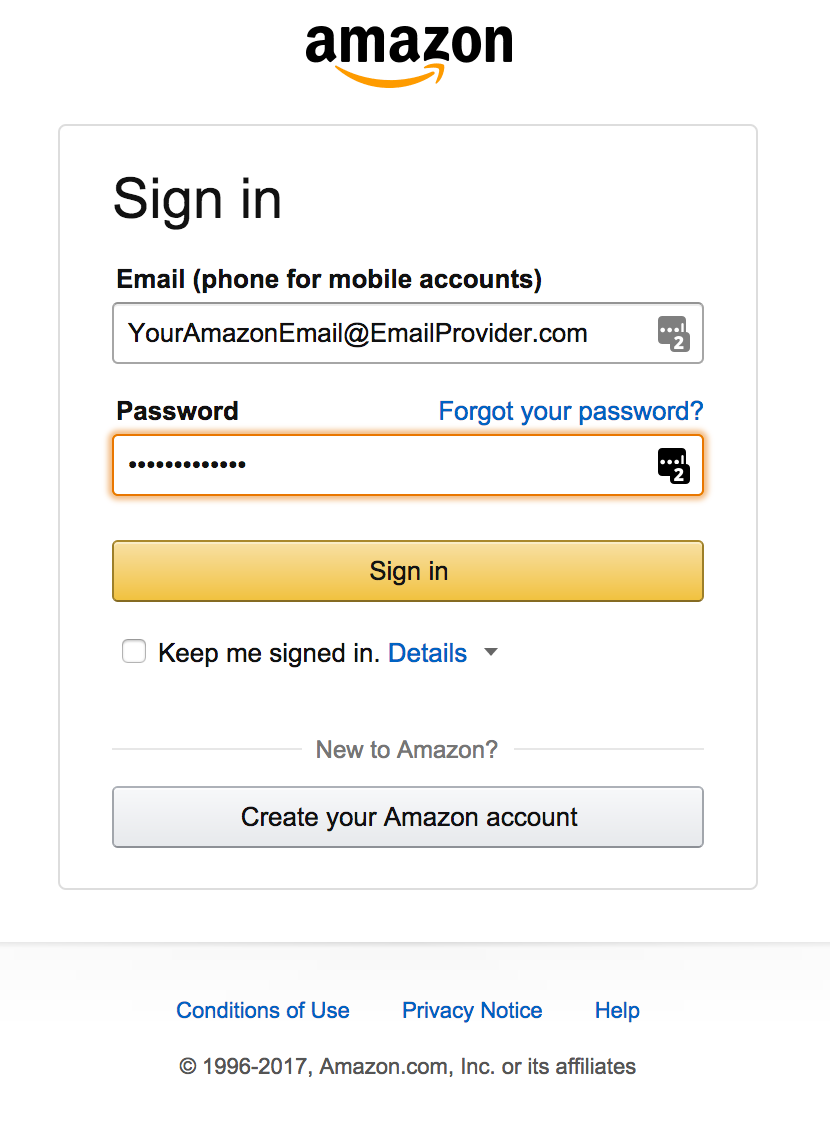The image depicts an Amazon sign-in page set against a white background. At the top of the page, the Amazon logo, featuring the iconic orange swoosh arrow, is prominently displayed. Below the logo, there is a white login box outlined in blue. The box contains fields labeled "Email or mobile phone for mobile accounts" with an example email address (yourAmazonEmail@example.com) shown in gray text. 

Additional fields include "Password" with an adjacent "Forgot your password?" link in blue. 

Below these fields, there is an orange "Sign-In" button and a small checkbox labeled "Keep me signed in" with a "Details" link followed by a downward arrow. 

For new users, there is a call-to-action link in blue that reads "Create your Amazon account." 

At the bottom of the login box are links to "Conditions of Use," "Privacy Notice," and "Help" in blue text. The footer of the page displays the text "© 1996-2017, Amazon.com, Inc. or its affiliates" in black print.